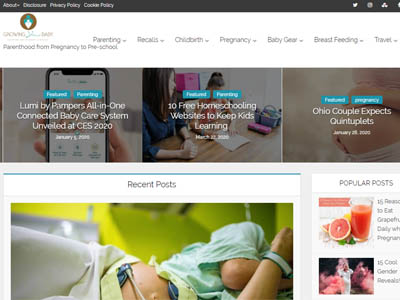The image is a small screenshot of a website designed in a magazine-style layout. Across the very top, there is a black bar, likely part of the browser interface, containing text that includes "About" with an arrow pointing right, alongside "Disclosure," "Privacy Policy," and "Cookie Policy." In the top right corner of this black bar, there are three white icons, although they are too small to be identifiable.

Below this bar, the main body of the website begins, set against a white background. In the top left corner, there is a logo or icon that appears to be a brown circle with a blue element inside. Directly below the logo, there is text that is difficult to read due to its small size, followed by the slogan, "Parenthood: From Pregnancy to Preschool." This text extends to the right and awkwardly flows underneath the navigation bar, which is positioned to the right of the logo. The navigation menu includes several drop-down options: Parenting, Recalls, Childbirth, Pregnancy, Baby Gear, Breastfeeding, and Travel.

Below the navigation bar, the website features three cover-image styled sections, each with a dark overlay and text, presumably previews of articles. The first section displays a person holding a phone and the text reads, "Lumi by Pampers All-in-One Connected Baby Care System Unveiled at CES 2020 January 1." The next section features two women on a hardwood floor with the text hinting at a free website for keeping kids engaged in learning. The final section shows an image of a pregnant belly with a woman's hands resting on it, accompanied by the caption, "Ohio Couple Expects Quintuplets."

Following these sections, the main content area is divided into two parts. On the left, there is a segment labeled "Recent Posts," topped by a large image that partially depicts a woman lying on her side in a hospital setting, with medical wires attached to her. To the right, there is a sidebar titled "Popular Posts," which displays previews of two articles, although the images are cropped, making it difficult to see them in full.